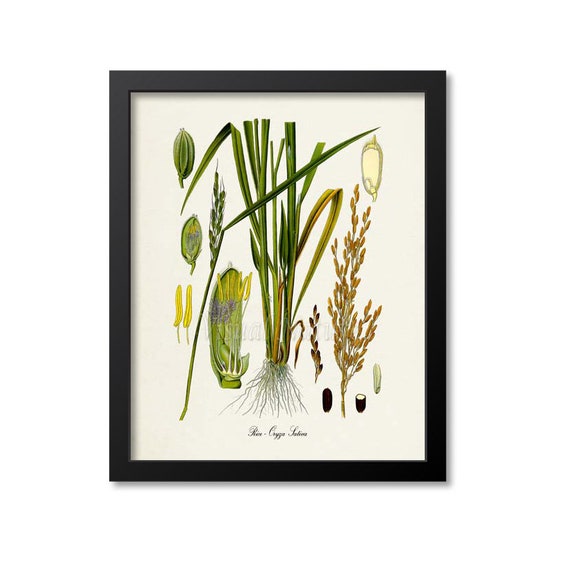A framed illustration, resembling a page from a vintage botanical book, depicts a detailed study of grassy plants and wheat-like specimens against a white background. The primary focus of the drawing is a central grassy plant with long, flexible stems that show its roots distinctly. Surrounding this central plant are various additional elements: on the right, smaller botanical components such as seedlings or cocoon-like pods, and a solid green structure that may have stamens. Also visible are individual parts that could be pistils and shafts of what appears to be wheat. The illustration is housed in a black frame, casting a slight shadow in the bottom right corner. At the base of the picture, cursive text is present but not legible, with an indistinct watermark also visible.